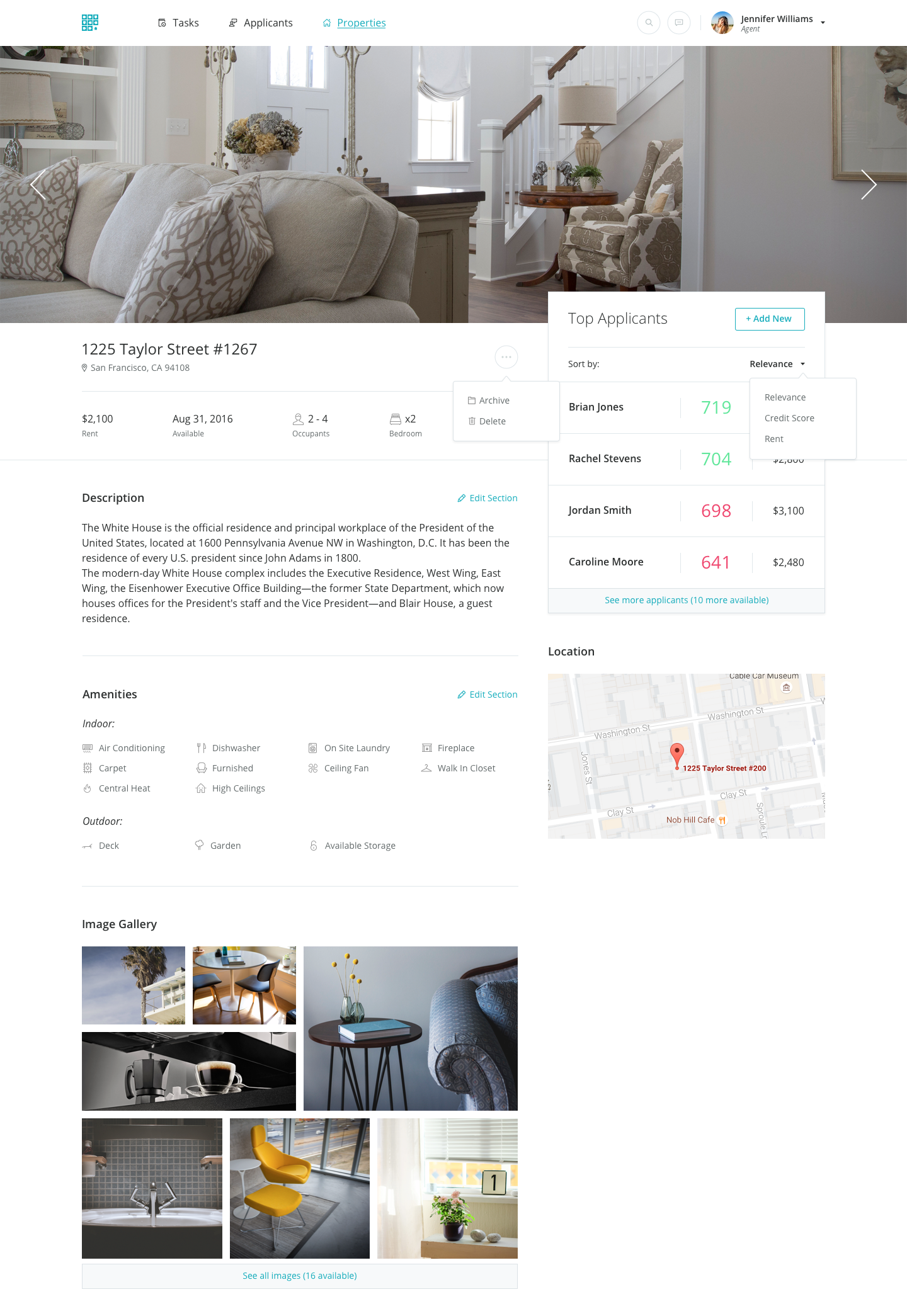This is a detailed screenshot of a real estate website interface. The background at the top is white, featuring a navigation bar with an icon displaying numerous squares arranged in a grid pattern. This bar includes the options for "Tasks," "Applicants," and "Properties," with "Properties" highlighted in blue while the others are in black font. 

In the upper right corner, the text "Jennifer Williams" is displayed alongside a small circular profile picture, though the image is too tiny to discern detailed features.

Below the navigation bar, there is a prominent photo depicting the interior of an exquisitely designed home, focusing on the living room and front door area. This room features pristine white walls and a largely white-colored palette. A beige couch adorned with throw pillows is positioned in the room, accompanied by lamps and a table with a basket of flowers, contributing to the room's elegant décor. The flooring is a light wooden hue, complementing the airy and bright ambiance. There is also a staircase leading upwards, adding to the homey yet sophisticated aesthetic.

Directly beneath the photograph, the text displays the address: "1225 Taylor Street, #1267, San Francisco, California 94108." Below this, a black separating line is followed by the rental details: "$2,100, available from August 31st, 2016," stating occupancy capacity of "2-4 occupants" and "2 bedrooms."

To the right of the image, a menu in a white square lists "Top Applicants." This section is sortable by relevance and includes the following names and scores: Brian Jones (719), Rachel Stevens (704), Jordan Smith (698), and Carolyn Moore (641).

There is also a brief and seemingly misplaced description about the listing, erroneously stating, "The White House is the official residence and principal workplace of the President of the United States," which does not align with the context of the listing.